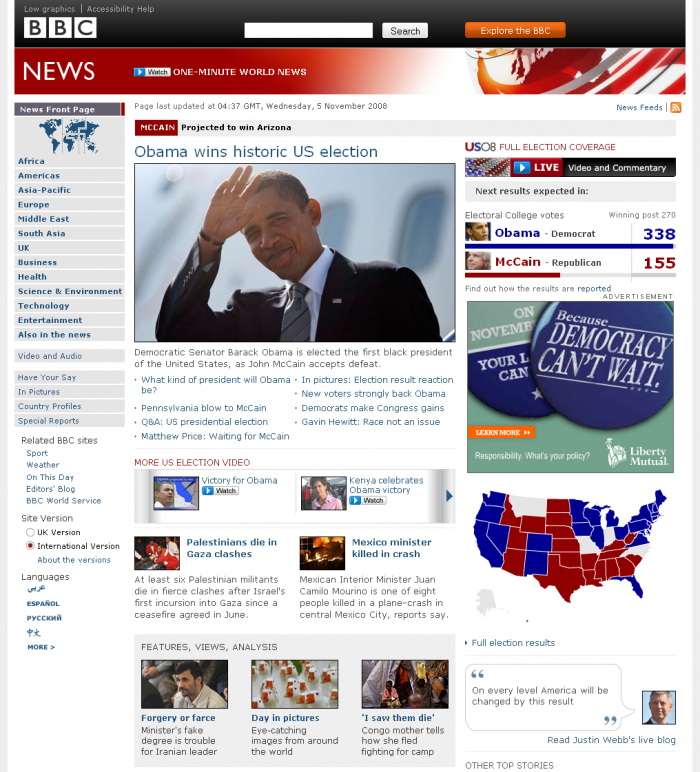This is a screenshot of the BBC News homepage from the day of Barack Obama's historic 2008 election victory. The central focus of the page is an image of President-elect Barack Obama, smiling and waving as he steps off an airplane. Directly beneath the image, a description reads: "Democratic Senator Barack Obama is elected the first black president of the United States as John McCain accepts defeat." Above this, a live news ticker announces, "McCain projected to win Arizona," emphasizing the ongoing election coverage.

Dominating the upper-right corner of the page is a poll showing Obama with 338 electoral votes compared to McCain's 155, vividly illustrating Obama's decisive win. An interactive map of the United States below the poll indicates the electoral results with states colored in blue, red, or gray to denote Democratic, Republican, and undecided outcomes, respectively.

The site's menu on the left-hand side provides navigation options, including links to various locations, categories, and related BBC sites. The page also features election-related advertisements from Liberty Mutual, underscoring the significant commercial interest in the historic event. Overall, the homepage is intensely focused on the 2008 election results, offering comprehensive coverage of Obama's landmark victory.